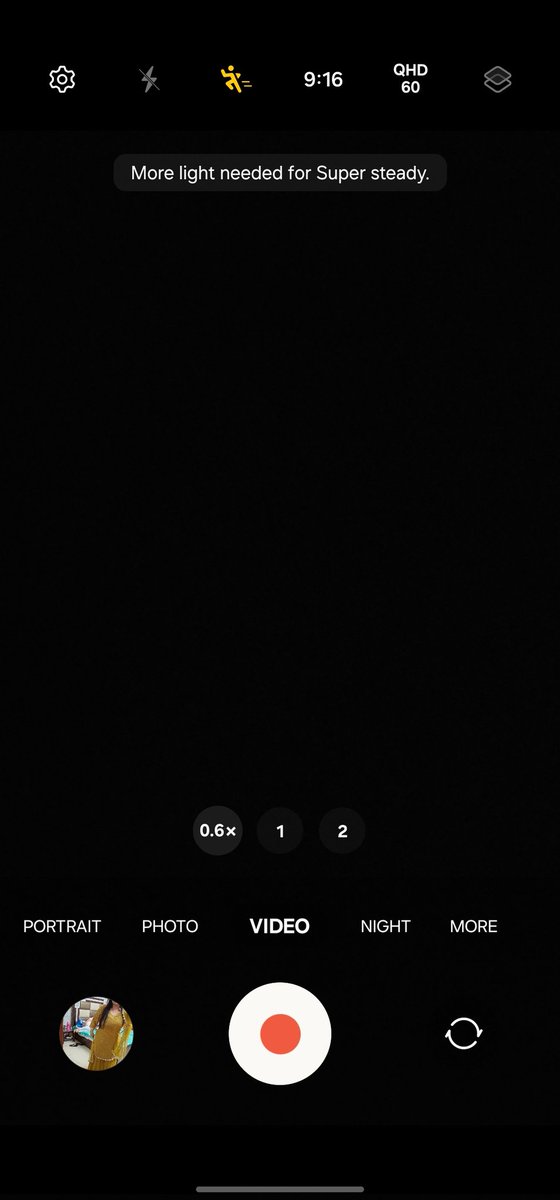"A striking image captures a woman in a shimmering gold dress, illuminated against a dark background. The scene exudes an electrifying energy, akin to a lightning bolt slicing through the sky. The photo, taken in portrait mode with a high resolution of 916 QHD, is composed of 62 meticulously stacked squares for enhanced detail. Despite the well-executed shot, more light might be needed for a super steady focus at 0.6x zoom. A gray refresh symbol and a record button are subtly visible at the bottom of the screen, with the rest of the space in deep black, adding contrast and emphasizing the elegance of the golden attire."